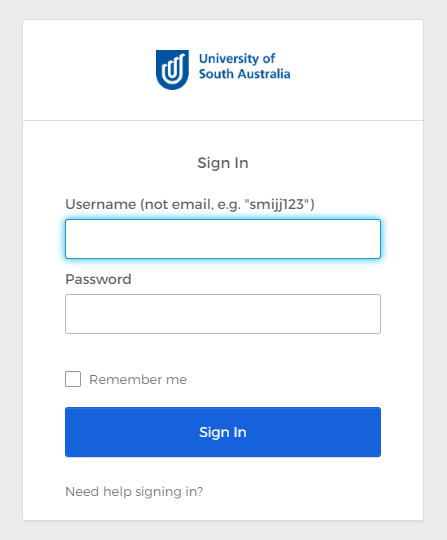The image depicts the login page of the University of Southern Australia’s website, which is characterized by a clean and minimalist design. The entire page features a pure white background, ensuring a sharp contrast with the university’s emblem and other critical elements in blue. 

At the top of the page, the University of Southern Australia's logo is prominently displayed in blue and white. The logo features a U-shaped design with a smaller U inside it. Directly beneath the logo, the text "University of Southern Australia" is clearly written.

Below the logo, the user is presented with a straightforward login form. The form starts with a "Sign In" heading. The first input required is a username, with a note specifying that it should not be an email address; an example username is provided for clarity. Following this is a text box where the username is to be entered.

Further down, the user must enter their password into another respective text box, preceded by the label "Password." Beneath this, there is a checkbox option labeled "Remember me," allowing users to stay logged in on the device. At the bottom of the form, a prominent blue "Sign In" button invites users to complete the login process. There is also a "Need help signing in?" link for users who might experience issues with the login.

The design uses blue sparingly but effectively, employing it in the university logo, the "Sign In" button, and the accompanying text, creating a cohesive and professional aesthetic. This login page is likely part of the main university website or accessed through an associated application, designed to facilitate access to student and staff accounts.